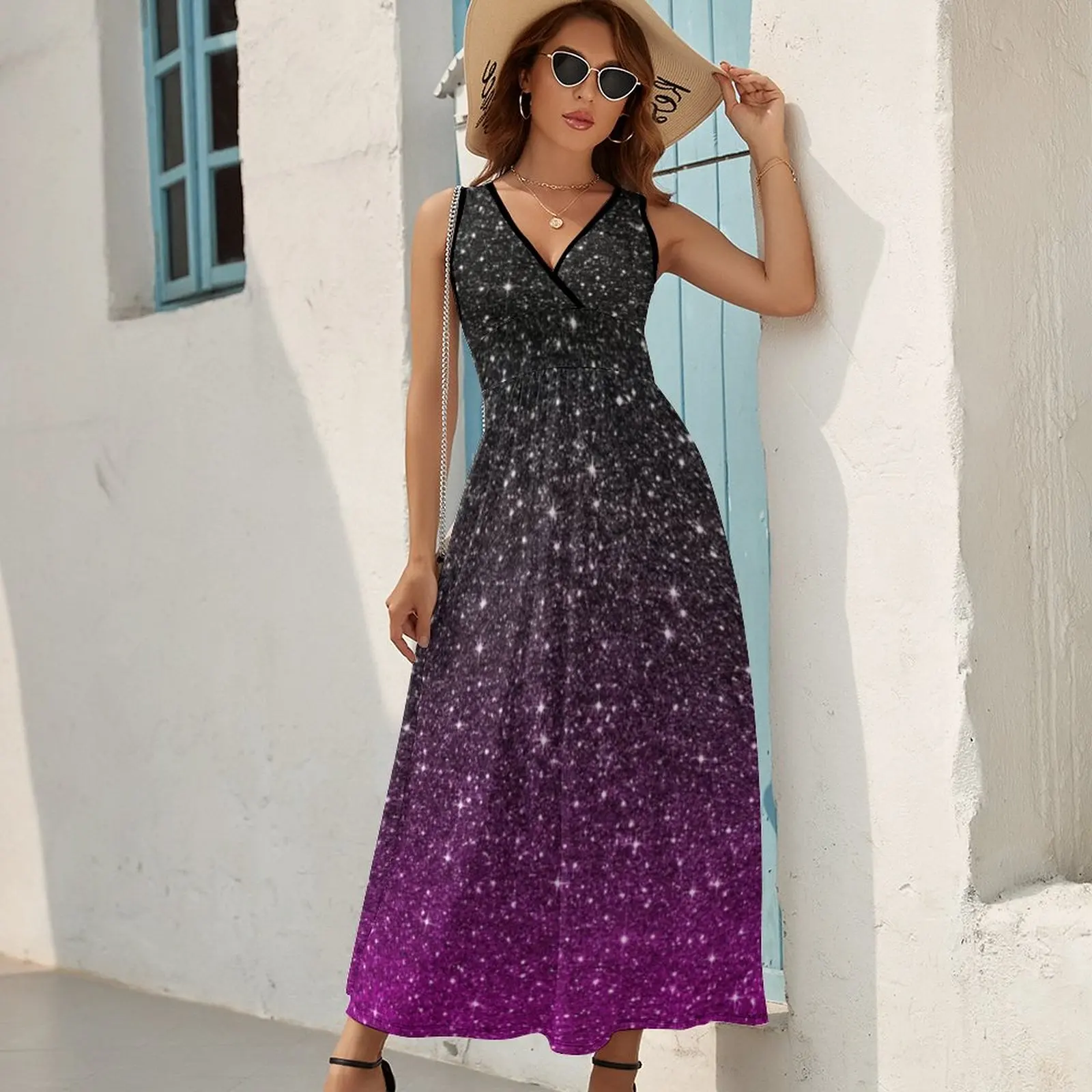In the image, a slender, very attractive woman is featured prominently, taking up the entire height of the picture and about 40% of the center width. She is dressed in a sleeveless ankle-length dress with a striking star field pattern, starting with a dark gray or black hue at the top, transitioning through dark purple, and ending in a lighter purple gradient near the hem. The dress appears to be adorned with sparkly elements, resembling a field of stars. She complements her attire with a wide-brimmed, floppy beige straw hat that has some unidentifiable black or navy text on the inside flap and stylish black sunglasses with white frames.

The woman has reddish-brown, wavy hair that falls to her shoulders and full lips accentuated with shiny pink lipstick. She accessorizes with two gold necklaces: a choker and another with a gold pendant. Carrying a small dark purse on her right shoulder, suspended by a silver chain, she strikes a confident pose with her left hand lifting or adjusting the brim of her hat while her right hand rests at her side.

Her footwear comprises black strappy high-heeled sandals, identifiable by the ankle straps encircling her legs. The background showcases a white stucco building bathed in natural sunlight, featuring a light blue wooden door directly behind her and a matching window to her left with blue shutters, adding depth to the scene. The overall composition exudes a stylish, summery vibe, likely intended to highlight the woman's fashionable outfit, reminiscent of a high-end fashion ad.